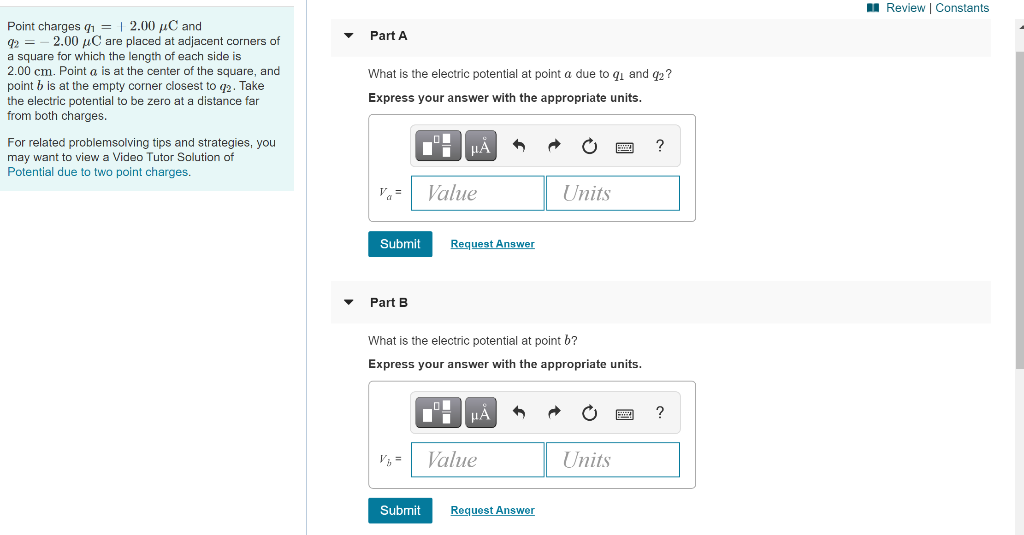This detailed image, taken on a smartphone or digital device, showcases a mathematical problem set against a bluish background. The problem involves electric potential calculations for point charges. Specifically, the problem states: "Point charges \( Q_1 = 2.00 \, \mu C \) and \( Q_2 = 2.00 \, \mu C \) are placed at adjacent corners of a square with each side measuring \( 2.00 \, m \). Point A is located at the center of the square, while point B is situated at the empty corner nearest to \( Q_2 \). Assume the electric potential is zero at a point far from both charges."

The problem further instructs: "For related problem-solving tips and strategies, consider viewing a video tutorial solution on potential due to two-point charges."

The problem is divided into two parts:
- **Part A**: Located at the top, it asks, "What is the electrical potential at point A due to \( Q_1 \) and \( Q_2 \)? Express your answer with the appropriate units." The answer field expects a value accompanied by units.
- **Part B**: Positioned at the bottom, likely asks for a similar calculation at a different point or under different conditions.

Both parts feature teal-colored options for submitting or requesting the answer.